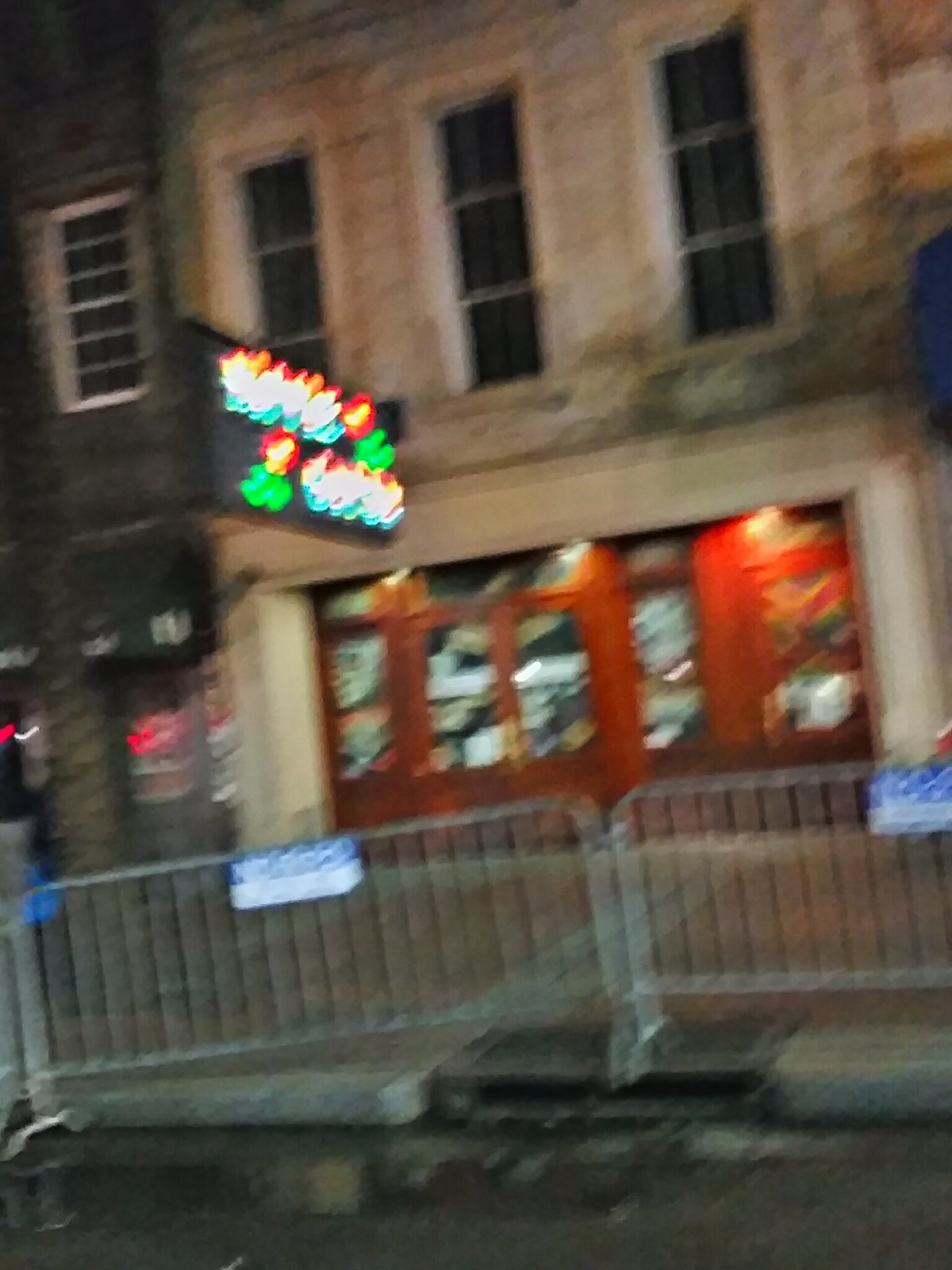This blurry image captures a street scene in a city, prominently featuring a pub or restaurant at the forefront. The building, likely made from stone or cement, has a striking exterior with high glass red doors and several windows on the ground floor, possibly framed by brown wood. Above these doors, there is a colorful, unreadable neon sign, with hues of yellow, green, white, and red indicated. The second floor showcases three long rectangle windows.

In front of the establishment, the sidewalk is marked by two metal guardrails, one of which leans slightly to the left, and they appear to be sections of barriers typically used by the police to manage crowds. Each guardrail has indistinct signs that are blue on top and white below. The sidewalk also features a drainage grate indicating some accumulation of water. Adjacent to this building is another gray structure with visible windows, possibly another business. The photograph appears to have been taken in motion, contributing to its blurry nature and making specific details hard to discern.